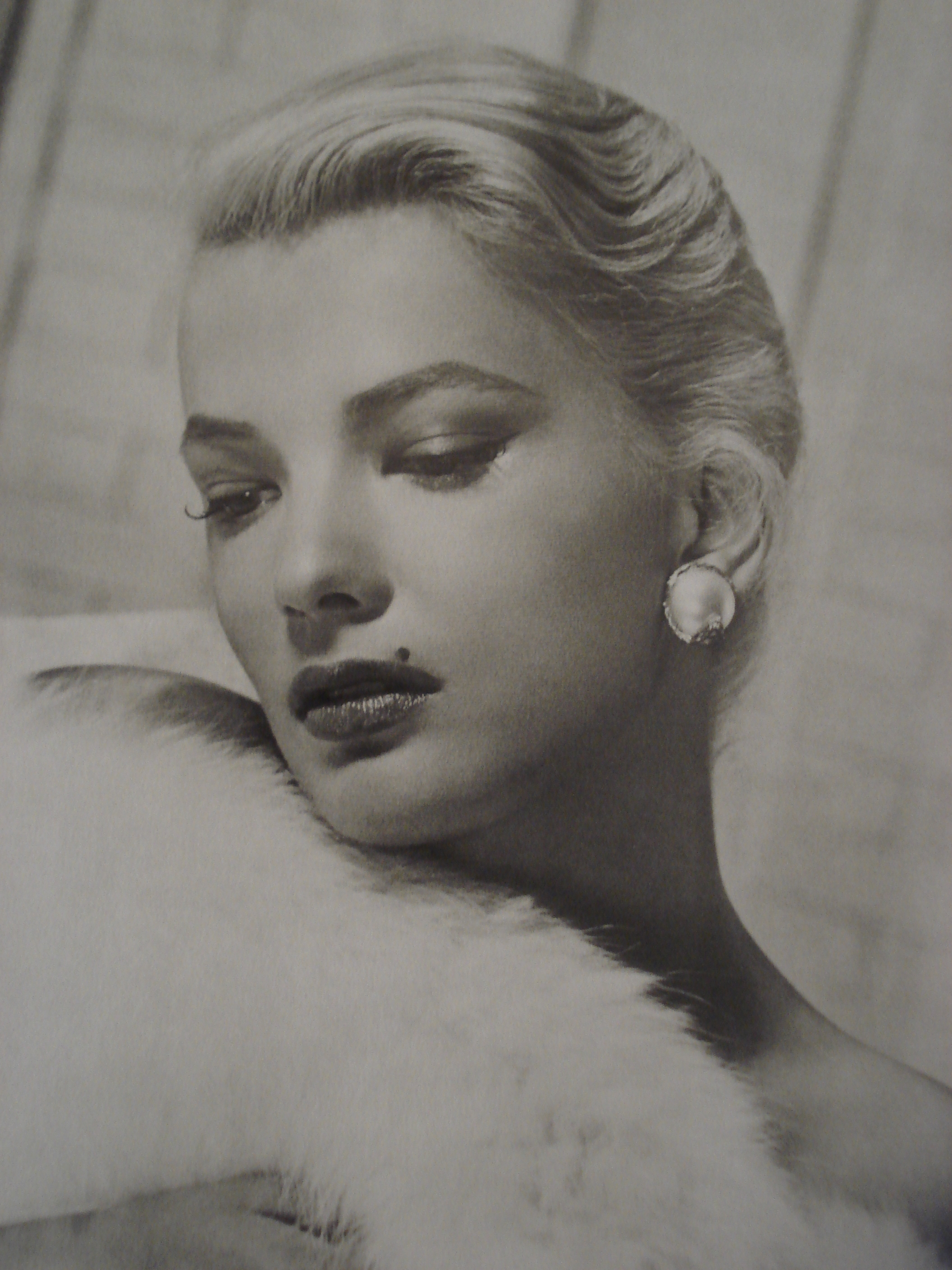The black-and-white image is a vintage-style headshot of a beautiful older actress or model. Her classy, wavy blonde hair is styled back, creating a medium-length appearance. She is adorned with large, circular jeweled earrings, of which only the one on her left ear is clearly visible. A distinctive mole is situated on the left side of her upper lip. Her makeup includes darkish eye shadow and meticulously curled long eyelashes, accentuated by her dark lipstick. The woman gazes seductively downward to the right of the camera. She appears to be holding or wearing a thick, luxurious fur piece that wraps around her neck and falls beneath her chest. The background is a white wall with vertical panel lines, adding to the sophisticated vintage ambiance of the photo.